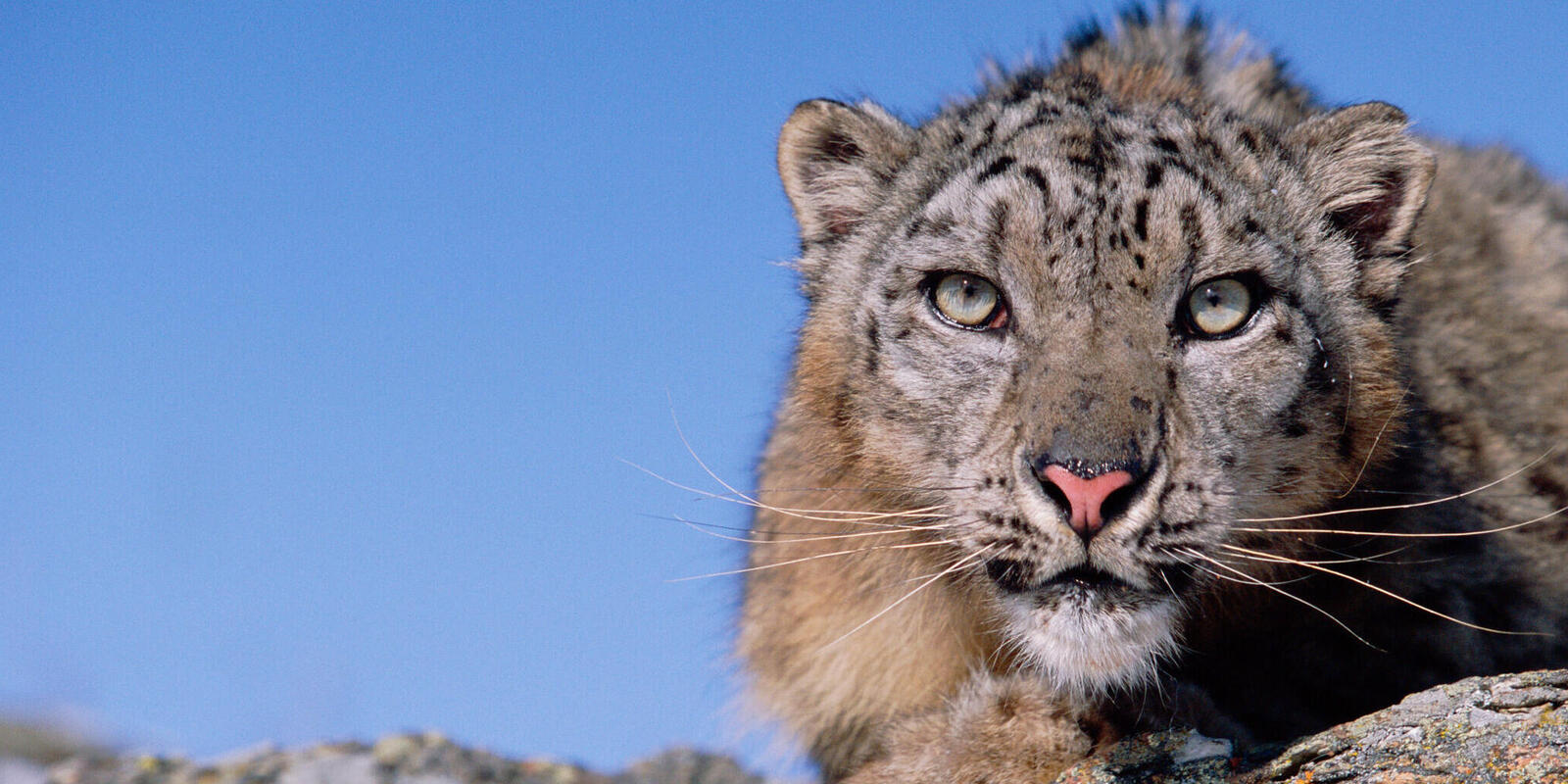A stunning close-up photograph captures the intense, piercing gaze of a snow leopard. The focus is primarily on the right side of the animal's face, highlighting its wet pink nose outlined in black and thick white whiskers jutting forward. The leopard showcases its distinctive tawny brown fur, speckled with black markings and a lighter white color around its face and under its mouth. The powerful eyes, a pale green with a fierce intensity, stare directly ahead, giving the impression of a vigilant hunter. The backdrop is a serene, slightly out-of-focus blue sky, complemented by a subtle glimpse of the rocky texture below, indicating the leopard's resting place. The animal's fur appears healthy, with no visible injuries, though there seems to be a small bite out of its left ear, adding character to its majestic appearance.